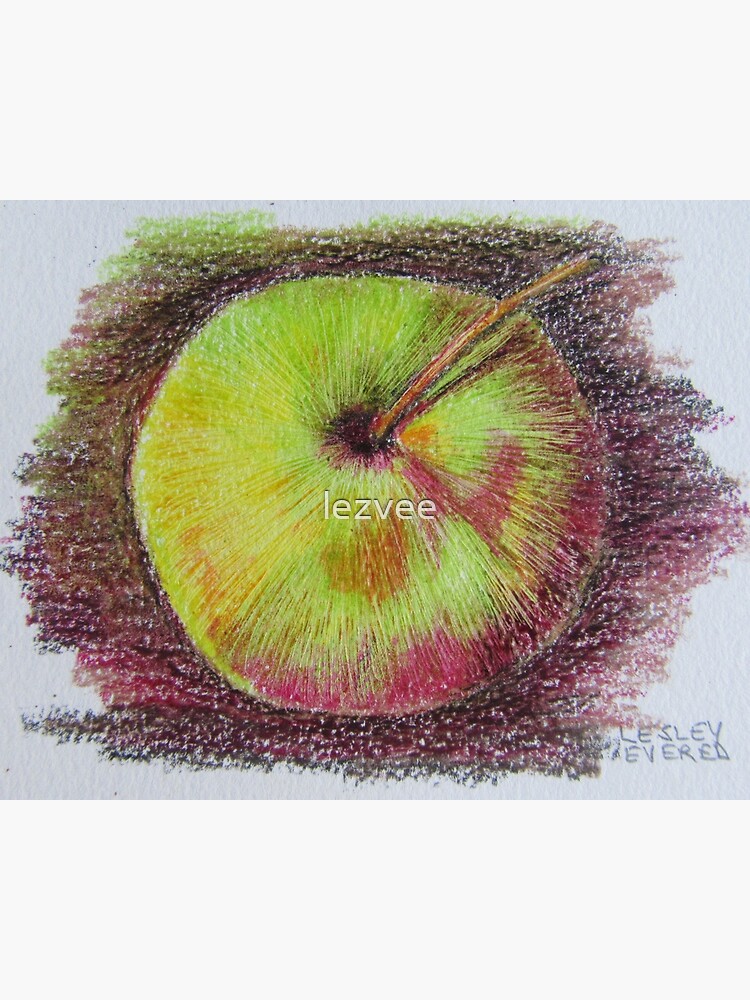The image displays a textured drawing of an apple viewed from the top. The apple, predominantly green with accents of red and orange, features a brown stem extending towards the upper right-hand corner. It appears to be created with pastels or crayons, employing strokes that radiate from the core, adding depth and dimension. The background combines hues of red and brown, resembling a dynamic abstract mixture of colors lightly smudged to support the apple. The artist's watermark, "Les V," is printed across the front of the apple, while the bottom right corner is signed "Leslie Everett." The entire piece is rendered on a textured, white paper surface, giving it an authentic, hand-crafted feel. The vivid shading and intricate use of color make this a captivating and well-rendered piece, likely available for purchase online.